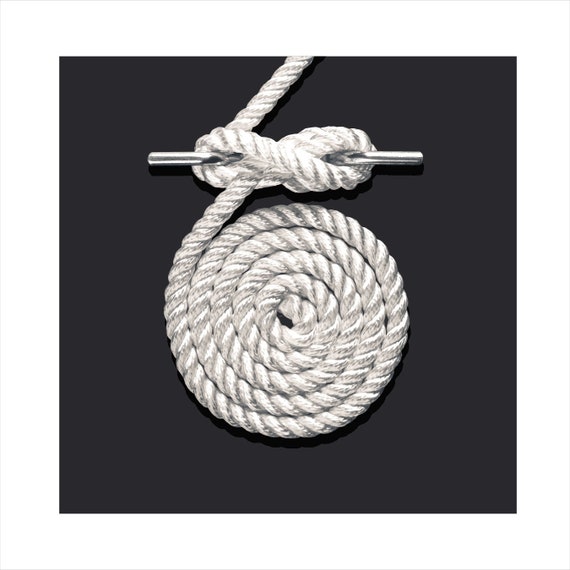This photograph features a meticulously arranged still life against a stark black background. At the center of the composition lies a length of white rope, artfully coiled in an intricate pattern. Just above the coiled rope, a slender, metallic object, partially wrapped in the rope in a figure-eight configuration, captures the viewer's attention. The metal object, reflecting ambient light, exhibits a mixture of silver and blackish hues, adding depth and contrast to the scene. Another segment of rope drapes over the top portion of the metallic element, casting a subtle shadow onto the black surface below, enhancing the interplay of light and shadow. Towards the center of the coiled rope, there is a slight blurring effect, drawing the eye to a small hole that offers a glimpse of gray through its opening. The image stands out for its excellent quality, showcasing the textures and details of the materials with precision.